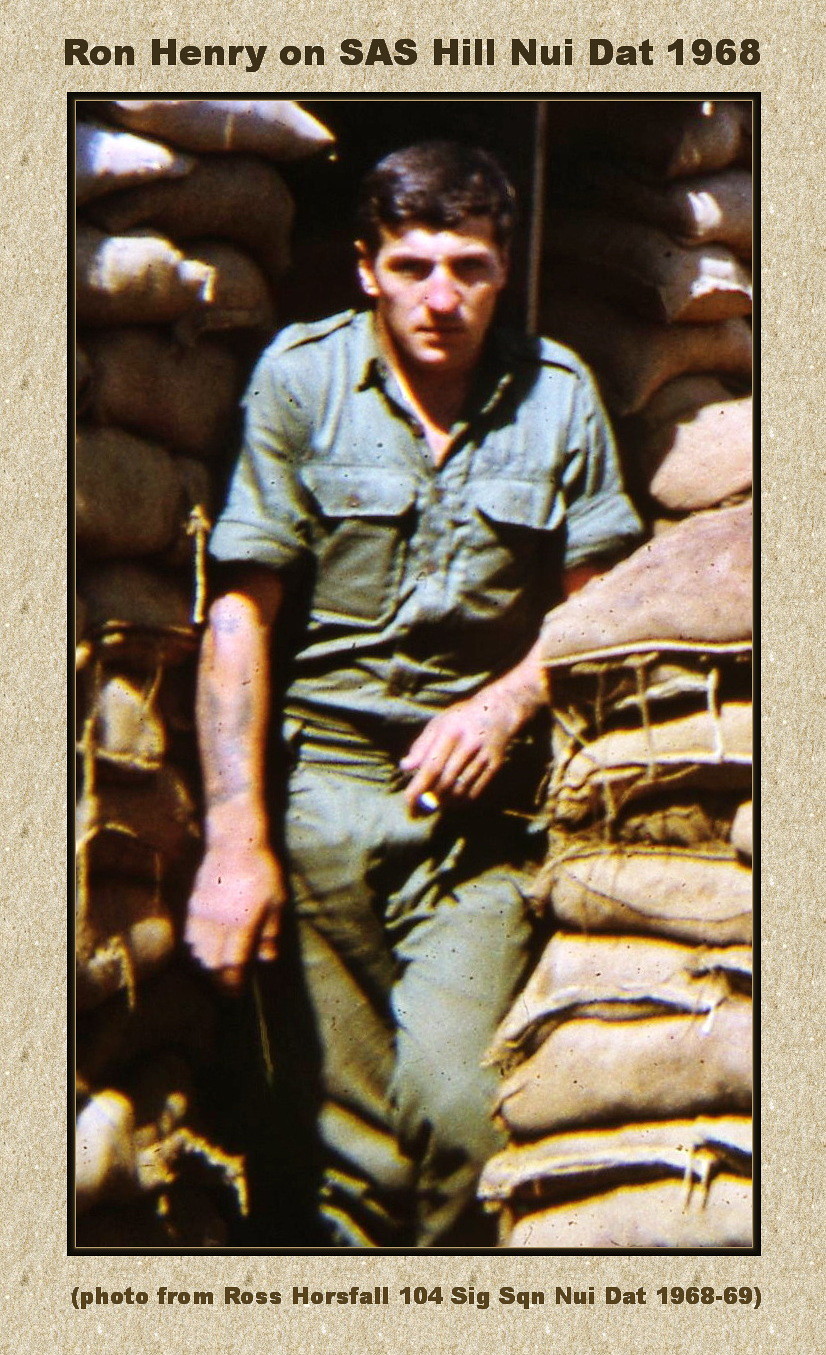The image is a vertically-oriented card with a light gray border surrounding a photograph at its center. At the top border, the text reads "Ron Henry on SAS Hill, Neudat, 1968." Beneath the picture, additional text notes, "Photo from Ross Horsfall, SIG Squin, Neudat, 1968 to 69." The photograph itself appears to depict a soldier standing outdoors in the daylight, likely set in Vietnam. He is positioned in the center of the image, facing directly at the camera. The soldier, who has short black hair and is clad in a green uniform, holds his right hand down at his side while his left hand is in front of his body. Surrounding him, particularly to his right, are stacks of sandbags or possibly grain sacks, which stretch from the bottom to the top of the image, creating a tan, brown, and green textured backdrop. The overall color palette of the image includes tan, brown, green, white, black, and gray, adding to the vividness and historic ambiance of the scene.